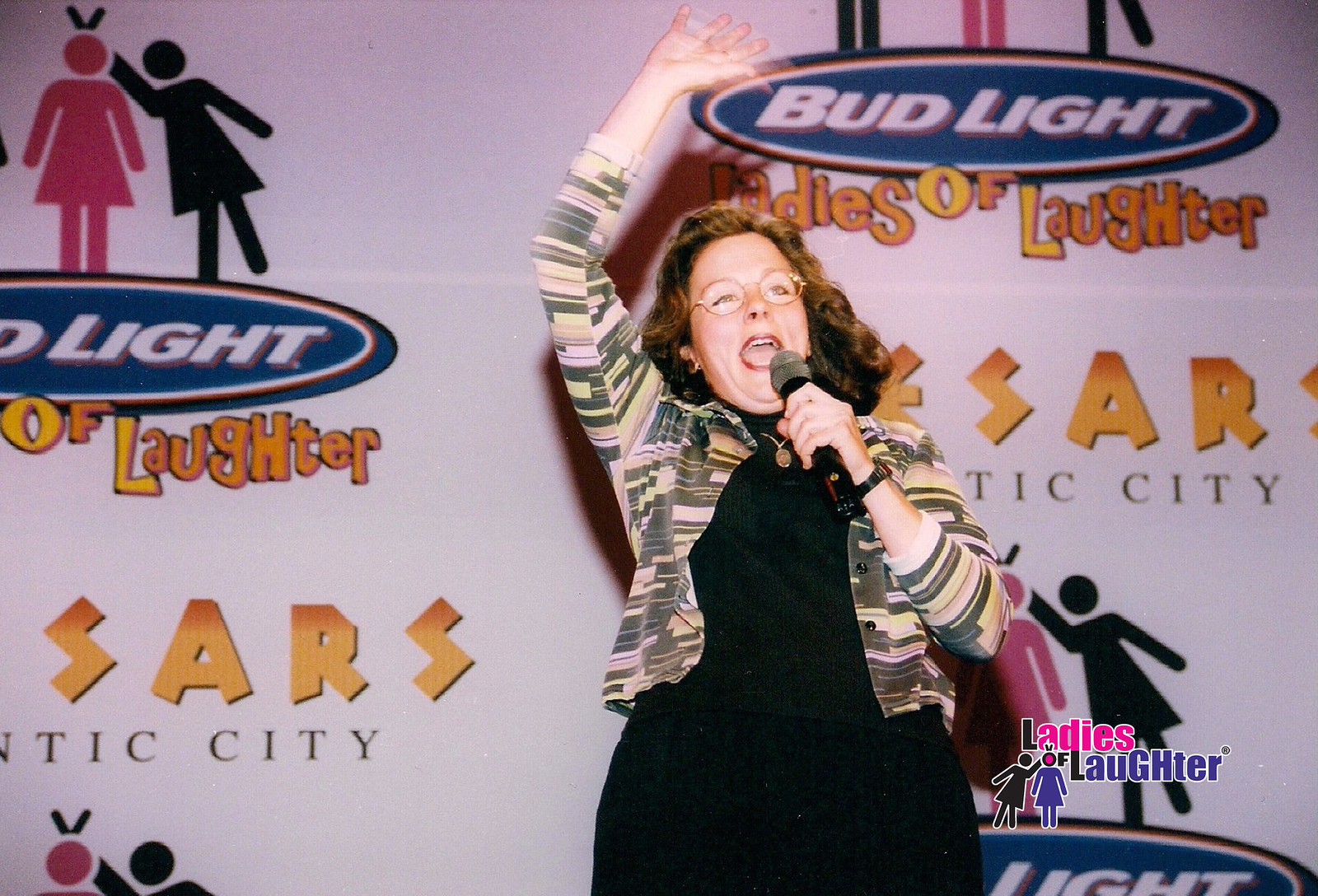In this image, a middle-aged woman with black and brown hair, wearing glasses and a wristwatch, is standing on a stage, holding a microphone in her left hand. Her right arm is dramatically extended high above her head, fingers splayed, as she speaks or performs. She is dressed in a black dress with a multicolored, geometric-patterned jacket that features shades of gray, black, beige, and white, ending just at her waist. Behind her, a backdrop is adorned with repeating logos and text. Prominently displayed at the top are the words "Bud Light" and "Ladies of Laughter" in a funky yellow-orange font. Below this, the name "Caesars Atlantic City" is visible along with images of three stick-figure-like women: a red one at the center, a black one on the right, and a less visible figure on the left. The overall scene suggests a lively stage performance or event dedicated to comedy and entertainment.